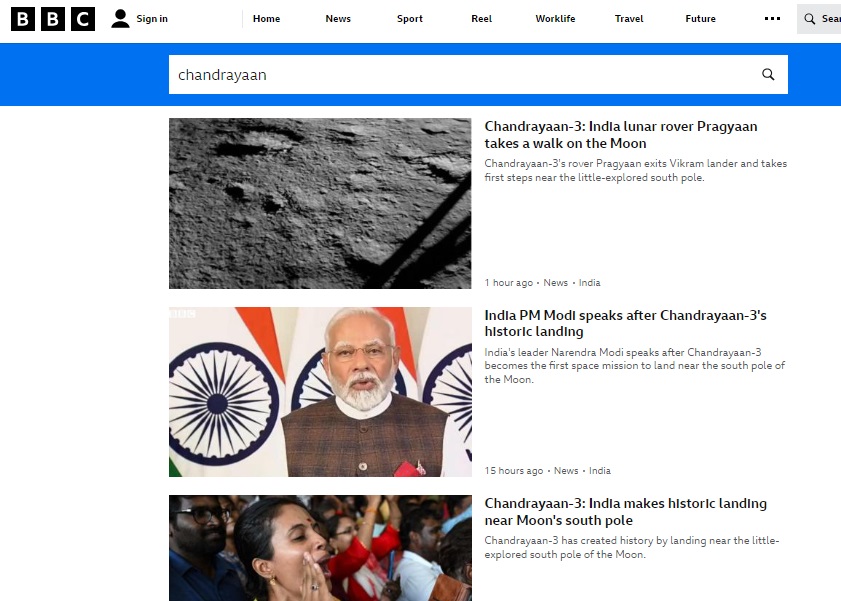The screenshot depicts a desktop or laptop screen displaying the BBC website. In the upper left corner, the BBC logo is prominently featured, with the letters "BBC" in white on a series of black squares. Next to the logo is a sign-in button. Along the top of the page, there are several navigation buttons labeled Home, News, Sport, Reel, Worklife, Travel, Future, as well as a More Options button represented by three black dots.

To the right of these navigation options is a search bar where the user has entered the query "Chandrayaan." The search results are displayed on a white background with black text. The first article result is titled "Chandrayaan-3: India lunar rover Pragyan takes a walk on the moon," detailing how Chandrayaan-3's rover Pragyan has exited the Vikram lander and begun its exploration near the moon's South Pole. The second article is "India PM Modi speaks after Chandrayaan-3's historic landing," covering Prime Minister Narendra Modi's remarks following the mission's successful landing near the moon's South Pole. The third article is titled "Chandrayaan-3: India makes historic landing near moon's South Pole," highlighting the significant achievement of the Chandrayaan-3 mission in exploring this less traversed region of the moon.